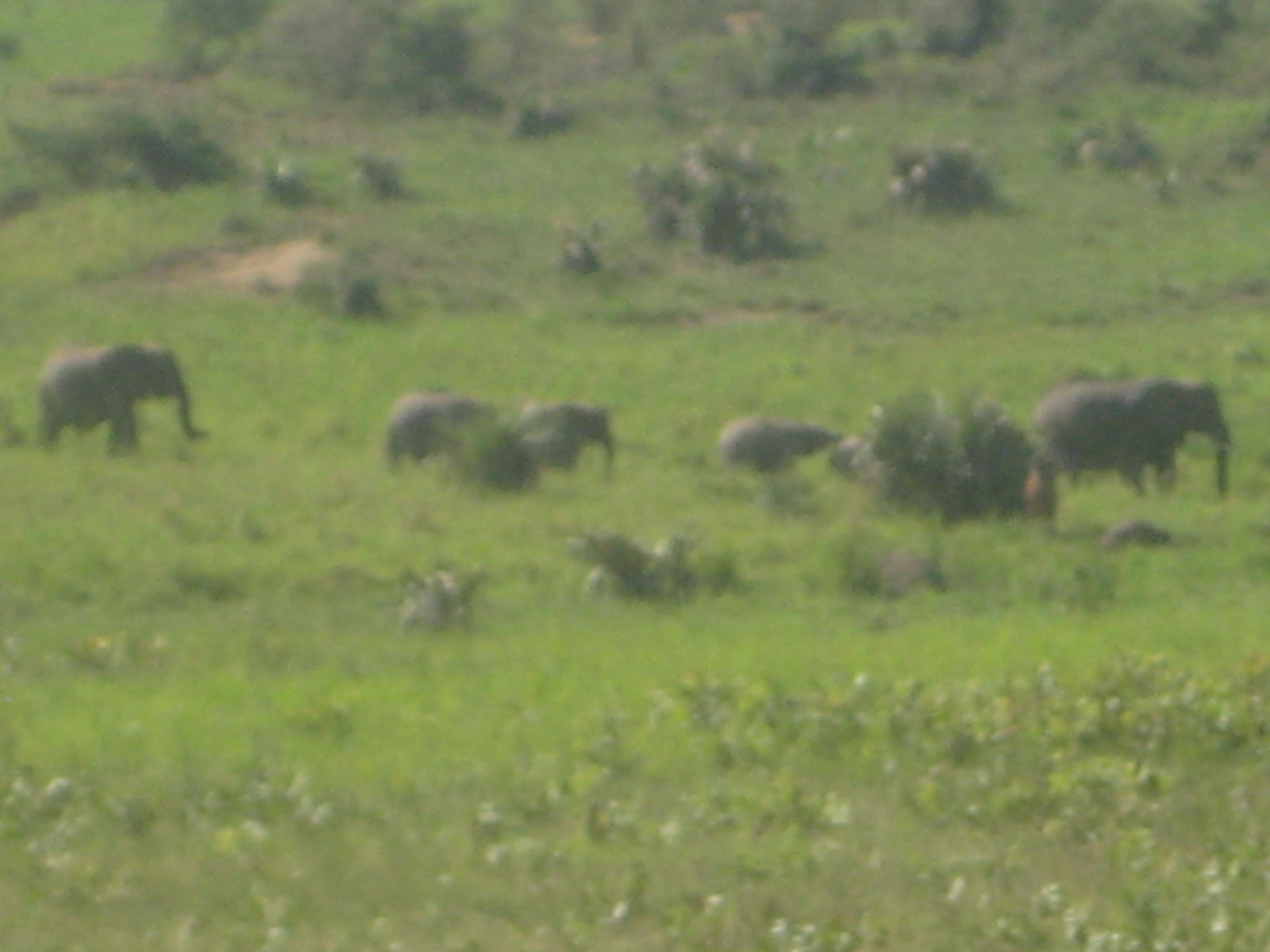The image depicts a distant view of a large grassy plain, possibly within a safari park or forested area, which features a family or herd of elephants. The scene includes several older and three baby elephants scattered around the lush, green landscape interspersed with shrubs and trees. Due to significant zooming, the image appears quite blurry and grainy, making it difficult to discern finer details or confirm if some distant shapes are elephants or rocks. The elephants seem to be going about their business, creating an impression of a natural, undisturbed setting. A small dirt spot can be seen on the left side of the field, adding to the image's serene and slightly unfocused ambiance.